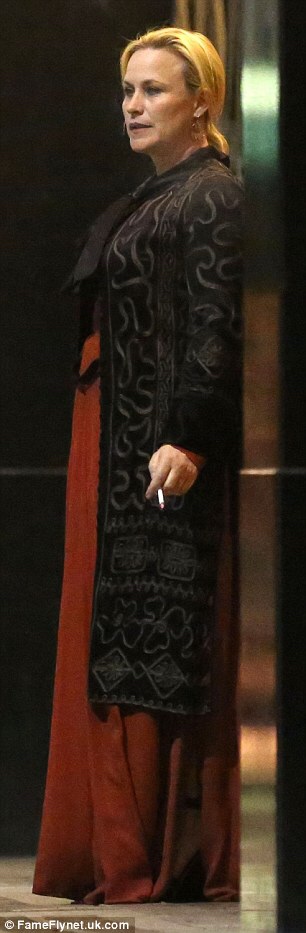This is a tall, narrow photograph of a woman, possibly Patricia Arquette, standing against a dark background with her back to the wall. The image, marked with the website fameflynet.uk.com at the bottom left corner, captures her in an elegant ensemble featuring a long, floor-length red gown and a stylish black overcoat adorned with intricate designs, which falls slightly above the gown’s hem. She has red or orangey-brown hair pulled back in a ponytail, and she appears to be in her 40s. The woman is holding a cigarette in her left hand, with her arm hanging naturally by her side, and is gazing off to the left. The scene is set on a gray floor and to the right of the image, there is a shiny, vertical section that suggests an elevator doorjamb. The photograph’s proportions emphasize its height over width, creating a striking and elongated visual effect. The background is predominantly dark with hints of green and a railing that hints at a lobby setting, perhaps just outside an elevator.